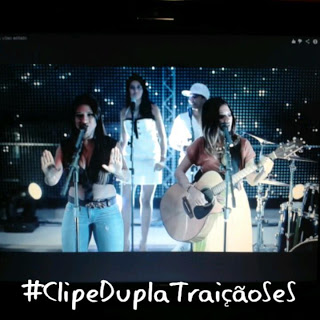A detailed photograph captures a band of four performers on stage against a black backdrop with a mesh fence and small, grid-like lights reflecting off it, creating a starry effect. The band features three women and one man. In the front, the lead singer, a woman with long dark hair, wears a sleeveless black crop top with a deep V-neck, exposing her midriff, and tight light blue denim jeans. Beside her, another woman with long dark hair strums a blonde acoustic guitar with a dark scratch plate. She sports an orange T-shirt paired with a light-colored skirt.

In the background, providing backing vocals, are another woman and a man. The woman at the back left wears a short white dress adorned with black accents, while the man next to her on the back right wears a white top, white trousers, and a white baseball cap. Both vocalists at the rear do not have visible instruments. At the bottom of the image, written in a handwriting-like font, is the hashtag: #ClipeDuplaTraicaoSES.